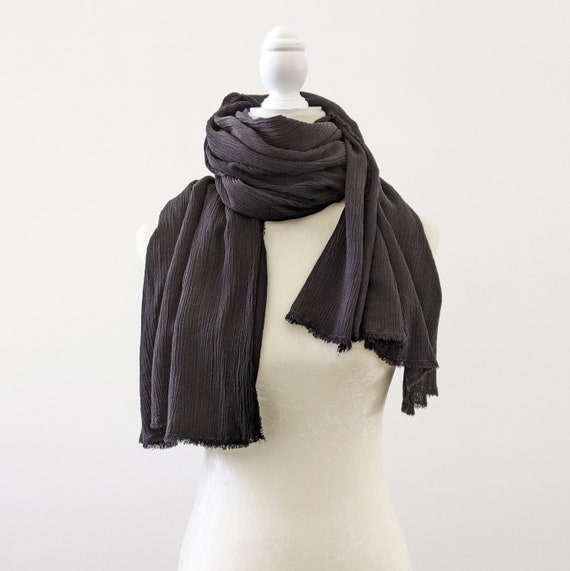This photograph features a square-shaped image with a plain off-white to light beige background that helps highlight the central subject: a white torso mannequin. The mannequin is smooth, round, and made of what appears to be plastic or cloth, suitable for pinning, with no head, arms, or defining characteristics besides a subtle white knob or egg-shaped top at the neck. Draped around the mannequin's neck is a crinkled, dark brownish-gray or nearly black scarf, which is lightweight and exhibits a crepe-like or gauzy texture. The scarf is wrapped around the mannequin's neck twice, with its edges neatly fringed and slightly frayed, falling down the front of the torso just about to the waist. The overall composition accentuates the contrasting shades of white and dark fabric, emphasizing the elegance of the scarf against the minimalist backdrop.